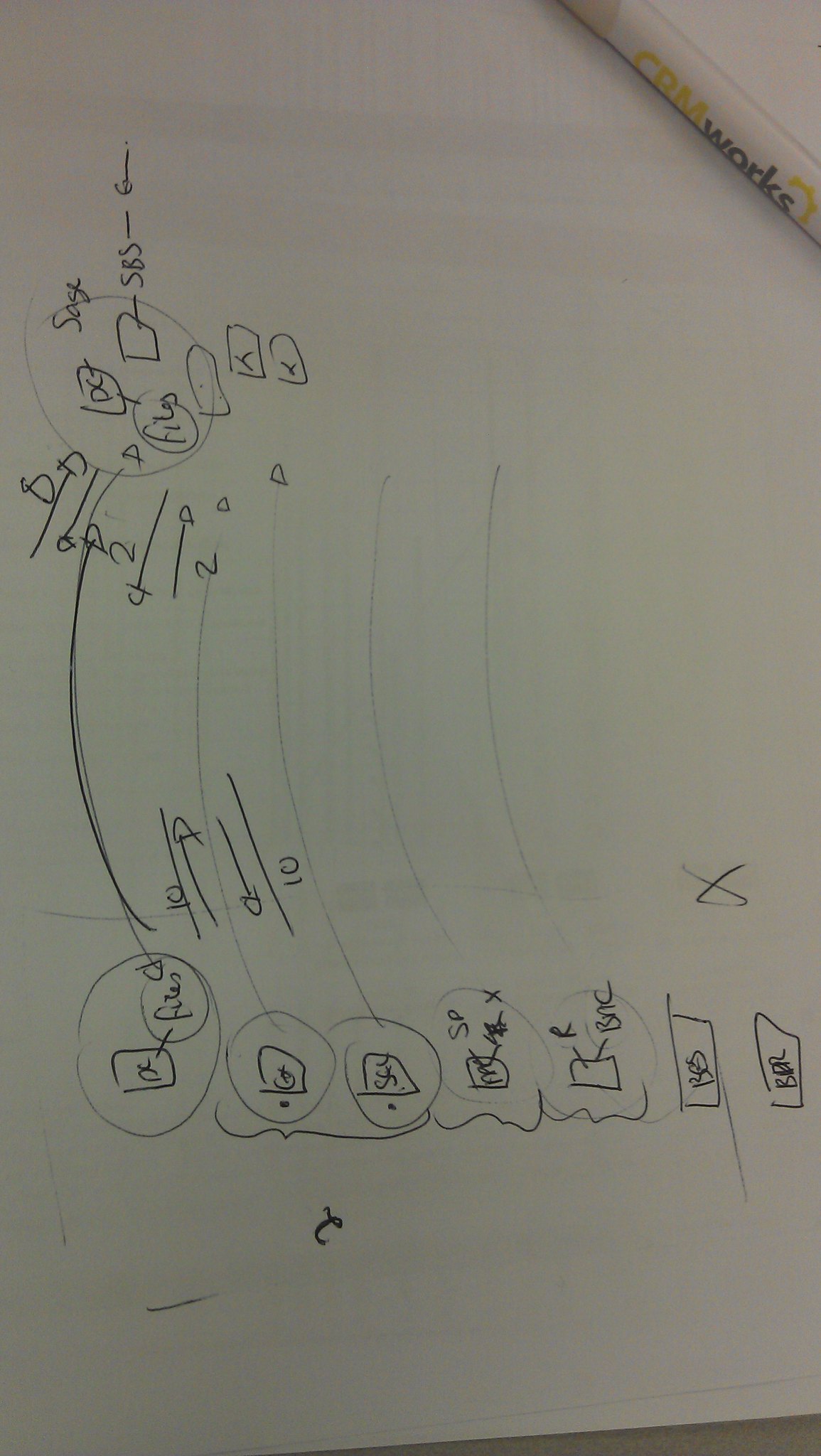Detailed Caption: 

In this photograph of a whiteboard, a detailed mechanical or electronic diagram is depicted with various shapes and symbols. On the far left side, there are two large circles connected by a long arrow, indicating some form of interaction between them. 

The top circle contains two rectangles and two components that appear to have an unusual design, possibly representing specific electronic parts. The lower circle features one smaller circle and one rectangle within it, potentially illustrating sub-components or processes.

Adjacent to the lower circle, there are two smaller circles, each housing a single rectangle, indicating further detailed sub-sections. Moving rightward, next to these smaller circles, are two rectangles positioned vertically, possibly denoting additional elements of the system, with what seem to be antennas protruding from the top, perhaps symbolizing wireless communication components.

Finally, on the far right side of the diagram, two more rectangles are present, each adorned with little squiggly lines in their centers, possibly representing resistors or similar electronic components. The precise interconnections and detailed representations suggest a complex system, possibly an electronic circuit or mechanical process being designed or explained.